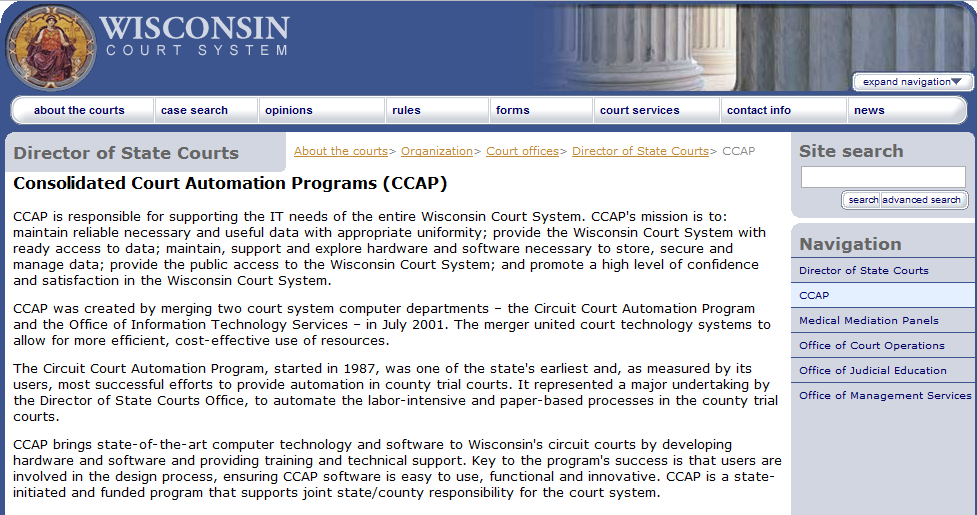The image is a horizontal, rectangular screenshot from a website, primarily featuring a white background. It includes a thin blue border on the left and right sides, with a thicker blue horizontal border along the top. On the right side of this top border, there are two close-up images of exterior structural columns. The left side of the banner displays a logo seal alongside the text "Wisconsin Court System."

Below the banner, there is a horizontal navigation menu on a white background, including options such as About the Courts, Case Search, Opinions, Rules, Forms, Court Services, Contact Info, and News. The largest part of the image lies below this menu and prominently features the titles "Director of State Courts" and "Consolidated Court Automation Programs," which go on to explain the CCAP (Consolidated Court Automation Programs).

On the right side of the lower section, there is a vertically aligned grey area dedicated to site search. It includes a search text window at the top. Beneath the search window, there's a vertical navigation list including options such as Director of State Courts, CCAP (which is highlighted), Medical Mediation Panels, Office of Court Operations, Office of Judicial Education, and Office of Management Services.